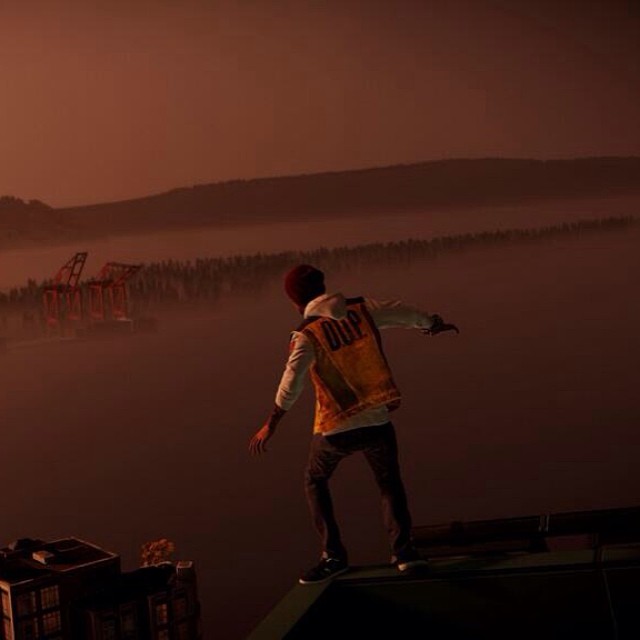This is a detailed screenshot from the video game series *Infamous*, likely from the second game, given the setting resembling Seattle. The sky is portrayed with a cloudy, tannish hue, creating a moody atmosphere. In the distance, a tree line and a mountain range can be seen. Prominent red cranes at a dock stand out against the landscape, denoting an industrial area. Below, several buildings with brown and white exteriors are visible. At the corner of one of these buildings, which features a green-colored ledge, a character stands poised. The character is distinctly dressed in a red cap, a white sweatshirt coupled with a yellow vest displaying the letters "D.U.P." on the back, gray pants, and black and white sneakers. The careful attention to detail in the character’s attire and the overall setting aligns with the game’s realistic and immersive design ethos.